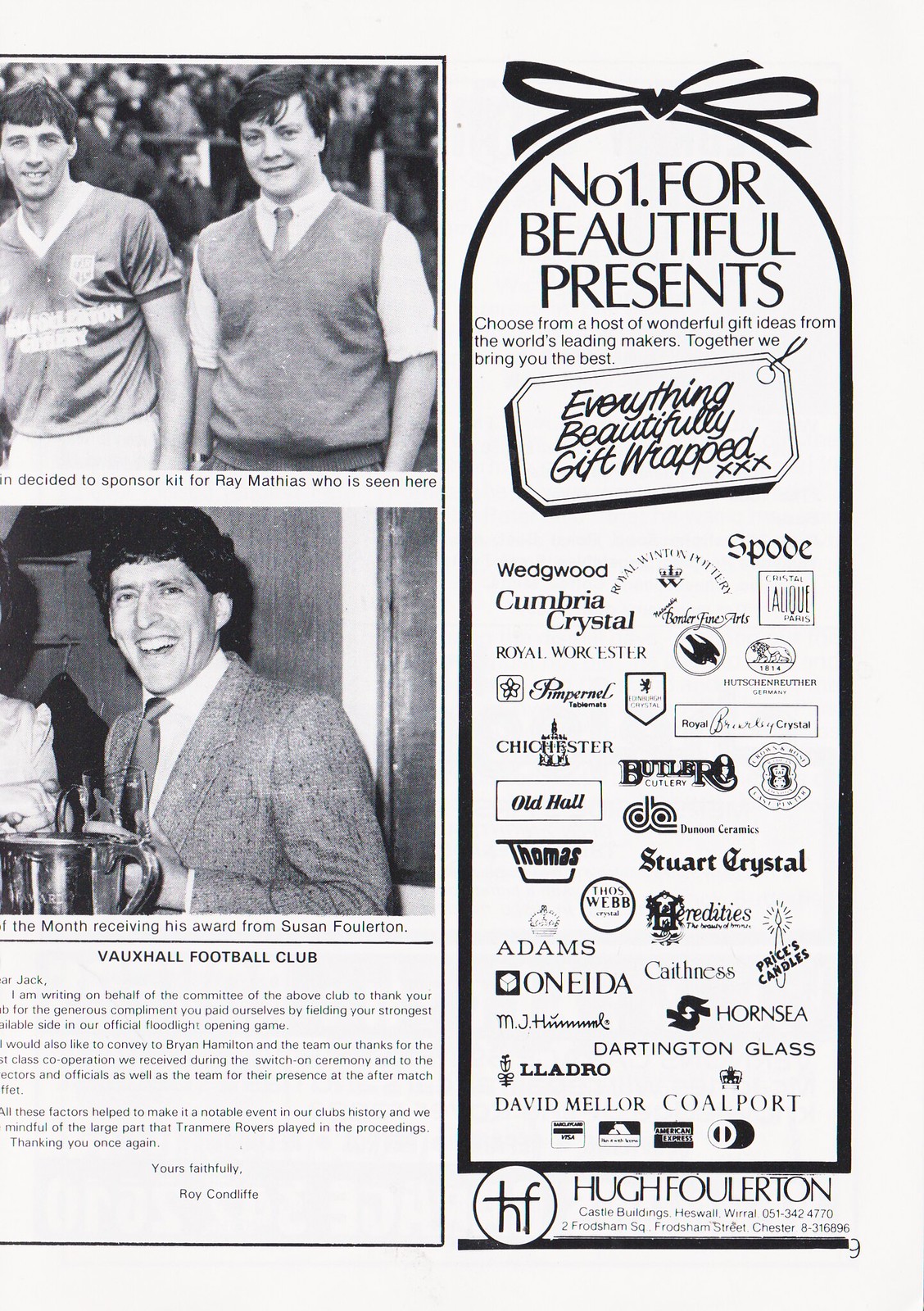The image depicted is a black-and-white page from a magazine, prominently featuring a banner and promotional content. On the left-hand side, two photographs are displayed. The first image shows a soccer player standing next to a young man in a school uniform, possibly depicting kit sponsorship for Ray Mathias. The second image below it features a man in a suit, smiling, standing next to a trophy, perhaps the same person from the first photograph. This man is identified as receiving an award from Susan Fullerton. Below these images, an article is titled "Vauxhall Football Club" with a letter signed off by Roy Condeff. 

On the right-hand side of the page, an advertisement with a thick black border and a decorative bow on top starts with the phrase "Number one for beautiful presents." The ad invites readers to choose from a variety of wonderful gift ideas from the world's leading makers, ensuring that everything is beautifully gift-wrapped. Several brand logos, including Cumbria Crystal, Royal Worcester, and Coalport, are listed within the border. At the bottom right, the advertisement features a logo labeled "HF" and the name Hugh Fullerton.